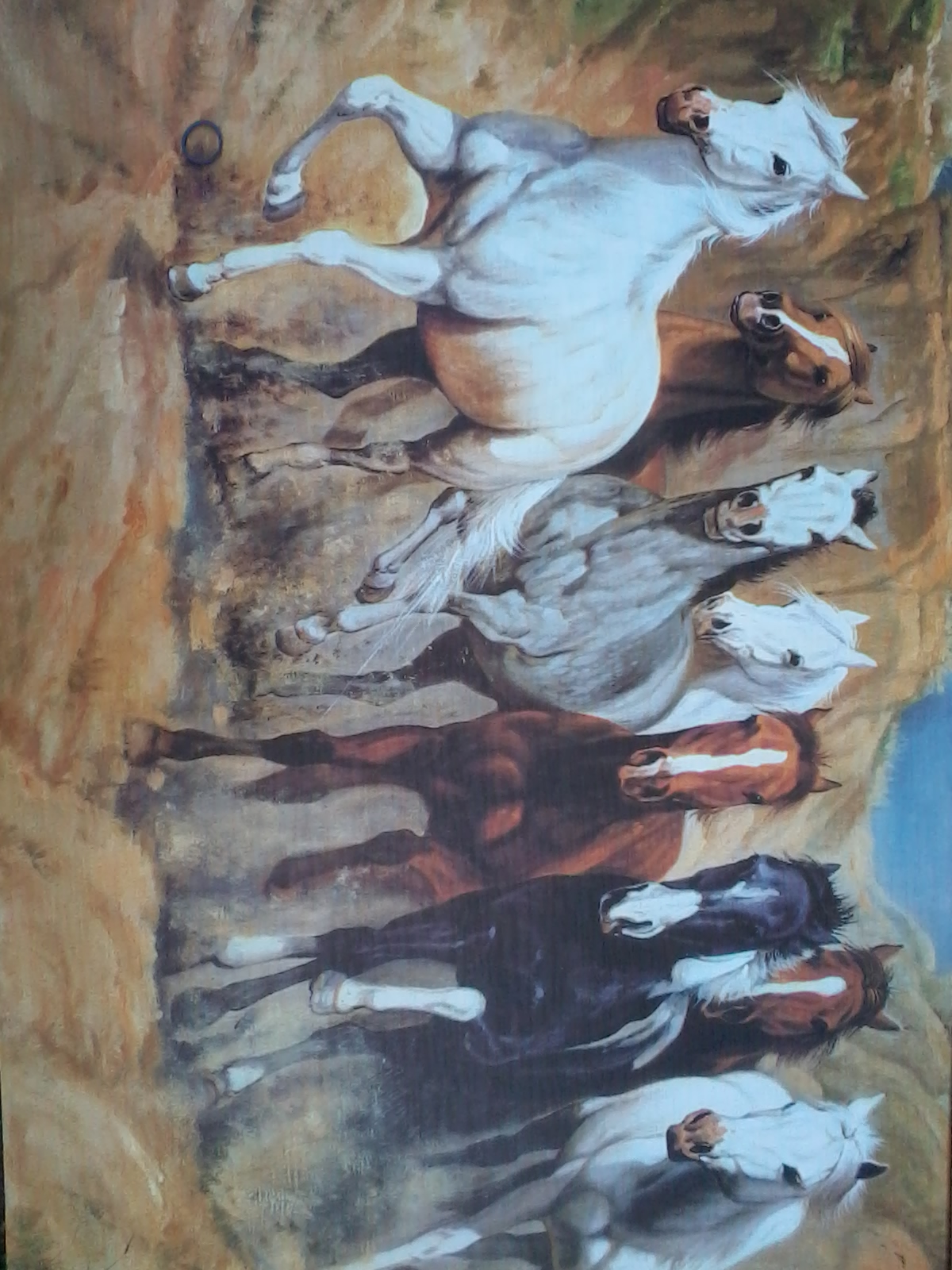This is a painting depicting a vibrant and dynamic scene of eight horses galloping towards the viewer. The painting is displayed vertically, although it was originally intended to be horizontal, giving it an unconventional perspective. In the foreground, a majestic white horse leads the group, its right front leg bent at the knee and its left front leg slightly off the ground, as it looks to the left. Next to it is a brown horse with a distinctive white stripe down the center of its face, with its mane flowing behind it. A third horse, white with a brown muzzle and black mane, shows hints of grey on its chest. Behind this horse, another white horse with a white mane can be seen. The painting also features a black horse with a grey nose and a white front hoof, captured mid-stride with its right hoof pushing off the ground. The final layer of the scene includes a white horse with a pinkish-brown nose and another brown horse with a white facial stripe, both appearing in motion. The background reveals a hint of blue sky above rugged, brown terrain, suggesting the setting of a canyon or gulch. The dirt ground beneath the horses and the wild setting underscore the freedom and energy of these magnificent creatures.